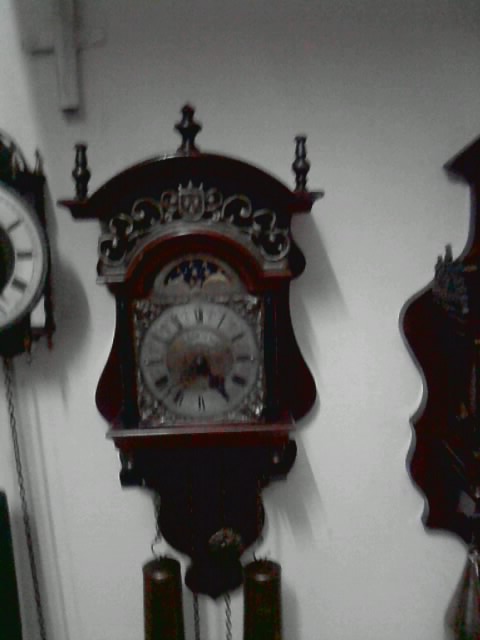This is a slightly out-of-focus photograph of a stunning European-made grandfather wall clock, believed to be from the 17th or 18th century. The clock, prominently displayed on a white wall alongside two other antique clocks, features a rich reddish-brown mahogany wood exterior and a sun and moon motif above the Roman numeral dial. The wooden structure has an arched top with darker mahogany pegs and a spindle design, capped with a leaf-patterned, crown-like embellishment potentially made of pewter. The silver clock face is adorned with swirls and black Roman numerals, with black minute and hour hands showing the time as approximately 4:43. Below the dial, two weights or pendulums, along with a chain, are visible, enhancing the antique charm of this exquisite timepiece.